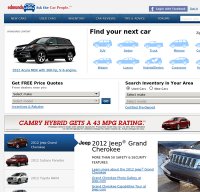This image showcases a webpage from Edmunds, a comprehensive automobile information website renowned for its extensive data and statistics on various cars. The focus of this particular page is car search functionality, enabling users to specify parameters like car type and year for targeted search results. Predominantly set against a clean white background, the webpage features a prominent blue banner at the top. This banner, adorned with white lettering, includes several navigational buttons for seamless user interaction.